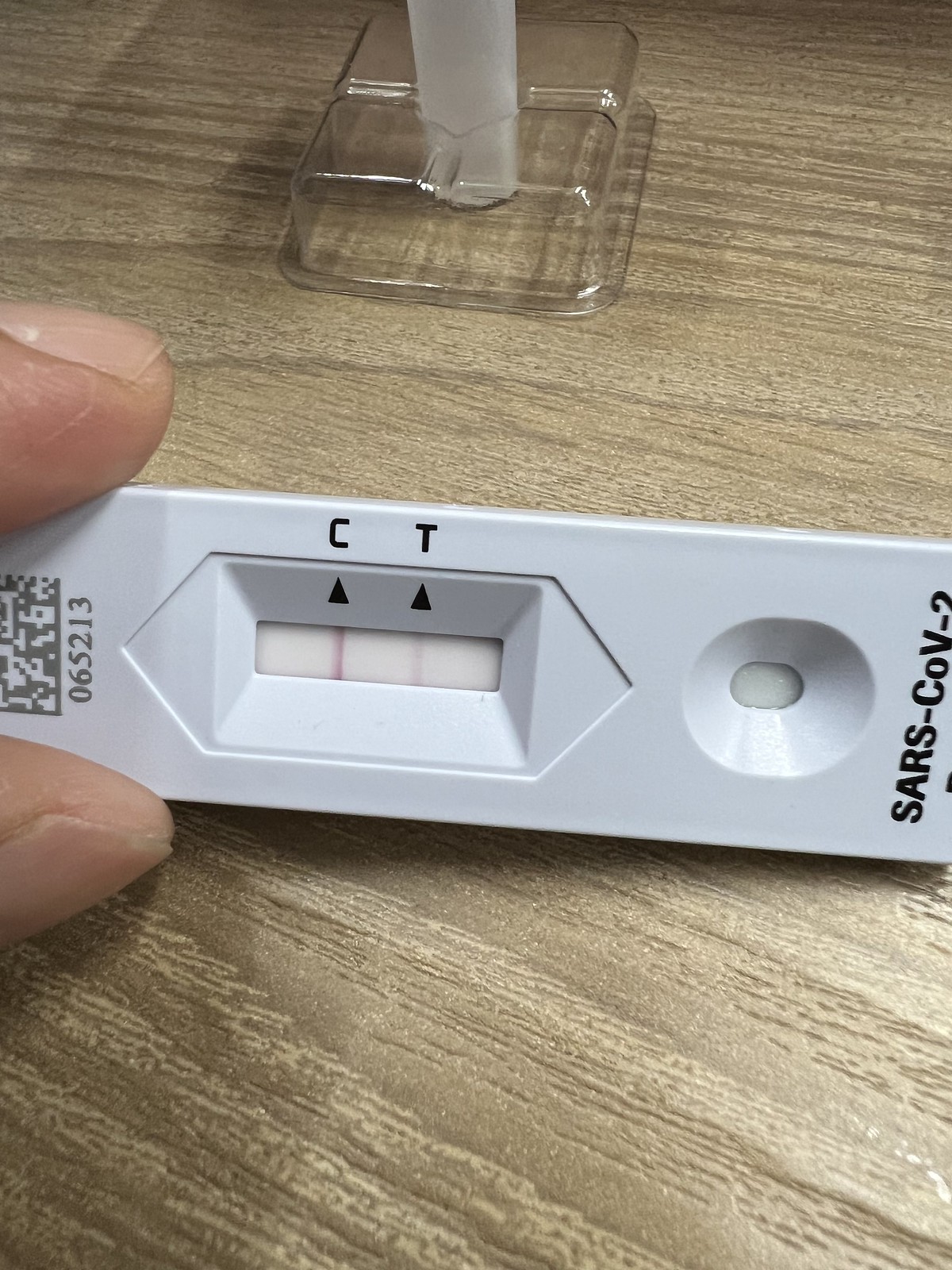The image is a detailed close-up of a SARS-CoV-2 rapid testing device. It shows the specific section where fluid has been recently applied, highlighting the areas labeled 'C' (Control) and 'T' (Test) with arrows pointing to their respective indicators. The test device is being held up by someone, just visible by the tips of their fingers on the left side of the image, against a surface that appears to be a light green wooden table. The result section clearly displays a dark pink line next to 'C' and a faint pink line next to 'T'. The presence of both lines suggests a positive test result.